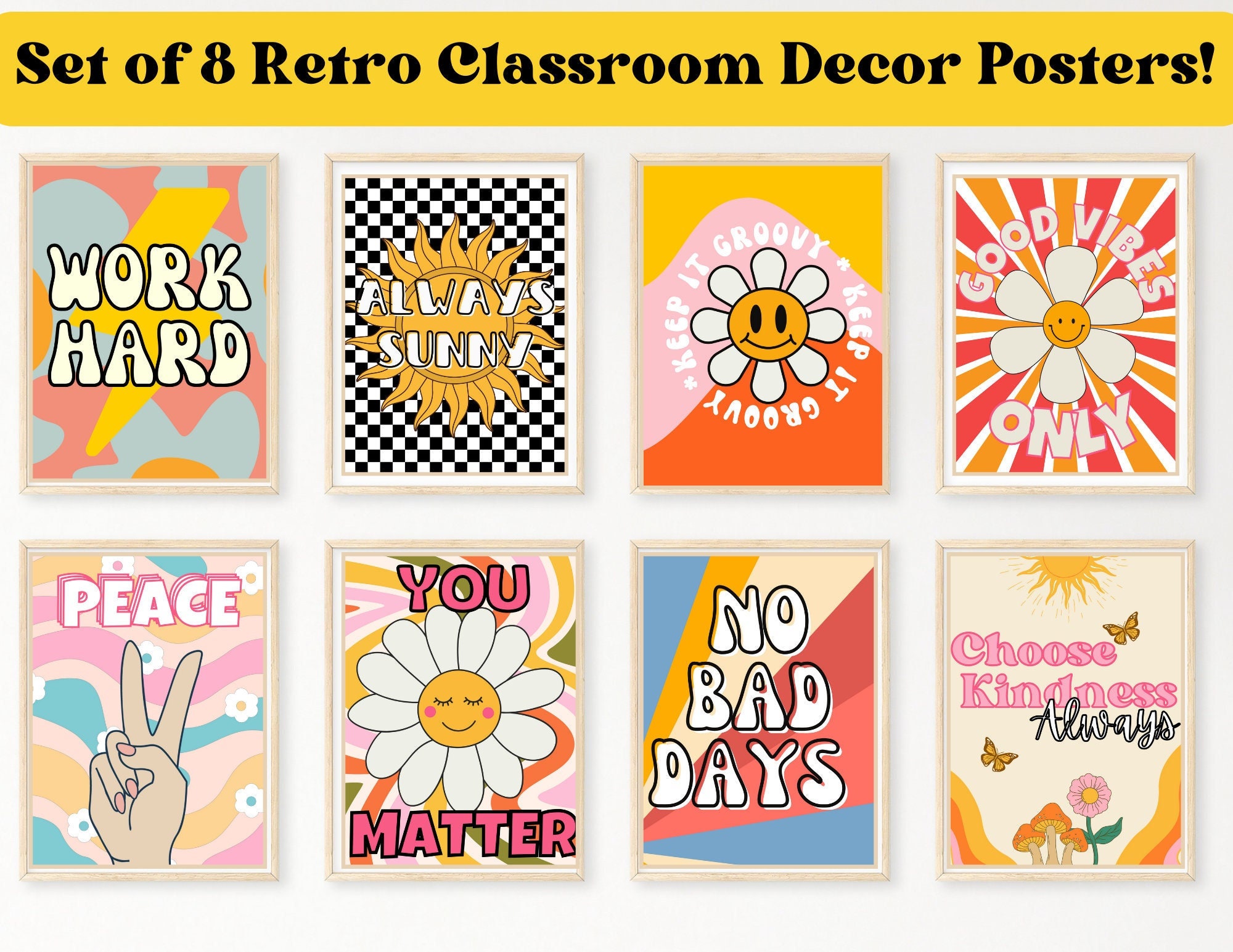This image showcases a set of eight retro classroom decor posters with a prominent yellow banner at the top reading "Set of 8 Retro Classroom Decor Posters" in black text. The posters are displayed in two rows of four and embody a groovy, hippie aesthetic reminiscent of the 60s and 70s peace movement.

In the top row, from left to right:
1. "Work Hard" - This poster features bubble lettering with a background of pink, gray, and a thick yellow lightning bolt.
2. "Always Sunny" - Adorned with a yellow sun at its center and a black-and-white checkered background.
3. "Keep it Groovy" - Showcases the phrase repeatedly in a circular pattern around a smiling daisy, against a colorful backdrop of yellow, red, and pink.
4. "Good Vibes Only" - Displays text around a six-petaled white flower with an orange smiley face and streaks of red, orange, and white radiating outward.

In the bottom row, from left to right:
1. "Peace" - Features a hand making the peace sign with nail polish, set against a background of red, pink, blue, and tan.
2. "You Matter" - Contains a smiling daisy with closed eyes, set amidst a swirl of yellow, pink, and white.
3. "No Bad Days" - Encapsulates the phrase in white letters on three lines, with a vibrant sunburst background of blue, orange, tan, red, and rose.
4. "Choose Kindness Always" - The phrase appears with "Always" in script, alongside illustrations of a sun, flower, butterfly, and mushrooms, against a tan background.

Each poster is distinguished by its vivid colors and cheerful illustrations, reinforcing themes of positivity, kindness, and peace.